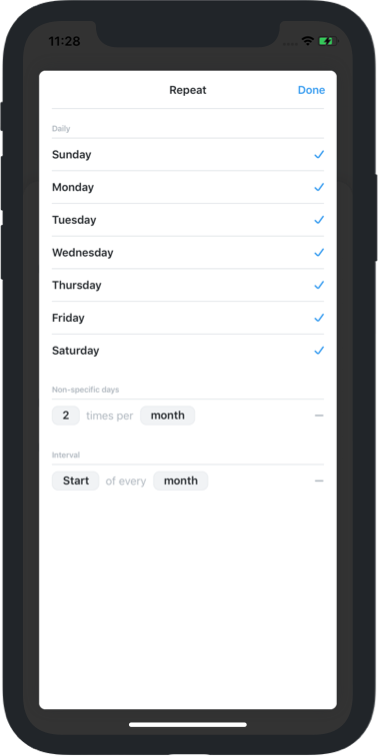The image showcases a smartphone screen displaying a to-do list or calendar application. The outer edge of the image features a dark gray frame emulating the shape of a smartphone, while a lighter gray border within it represents the screen. In the top-left corner of the screen, the time is displayed as 11:28. In the top-right corner, there is a Wi-Fi icon with full signal strength (three out of three bars) and a battery icon that is approximately three-quarters full and green, indicating a partially charged battery.

The main interface has a white background with the title "Repeat" prominently displayed at the top. Next to the title, the word "Done" is highlighted in blue. Below the title, the screen is divided into two main columns. The left column lists various frequency options, starting with "Daily." Each day of the week from "Sunday" through "Saturday" is mentioned, and the corresponding right column shows a series of blue check marks under the "Done" heading, indicating completion.

Further down the screen, there is a section for non-specific days with an entry labeled "Two Times Per Month" followed by additional options. The bottom section allows for selecting intervals and specifies the start of every month, which has been selected by the user. Overall, the image provides a detailed view of a well-organized repeat task scheduling interface on a smartphone.